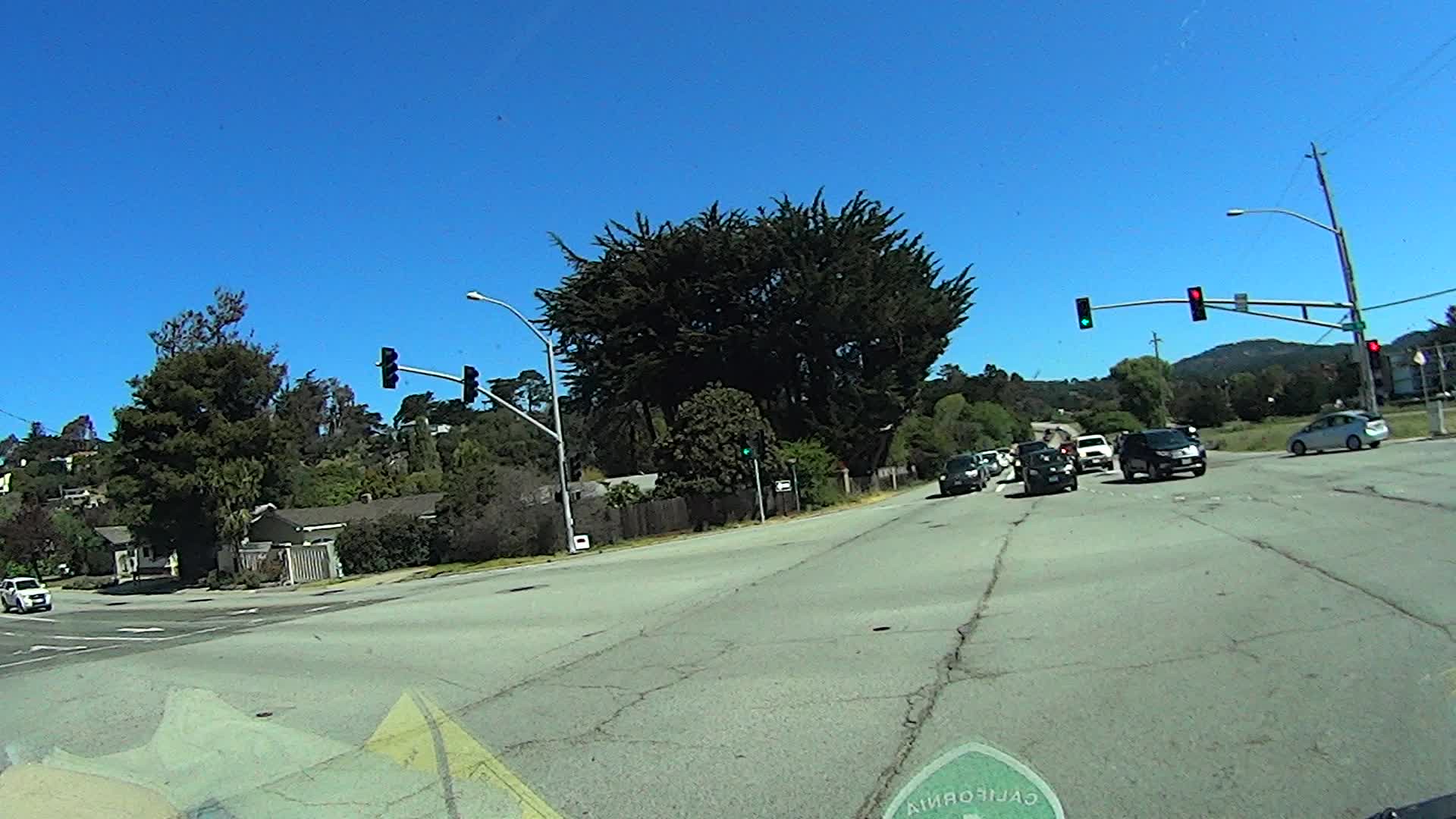This daytime photo captures the view from inside a car, looking out through the front windshield at a bustling intersection. The scene is filled with several cars, some moving and others stationary, reflecting a moment of traffic activity. The intersection features a set of traffic lights visible directly ahead: a green left-turn arrow and a red light for going straight. The bright blue sky, completely free of clouds, suggests a clear summer day. Low houses and tall green trees are partly visible along the sides of the scene, adding to the suburban feel. Interestingly, there are markings on the pavement that appear as a mirror image, hinting that the picture might have been reflected; one text seems to read "California," associated with a shield-like shape resembling a road sign. The photograph, taken in portrait orientation, captures the essence of a sunny and vibrant day at this busy Californian intersection.